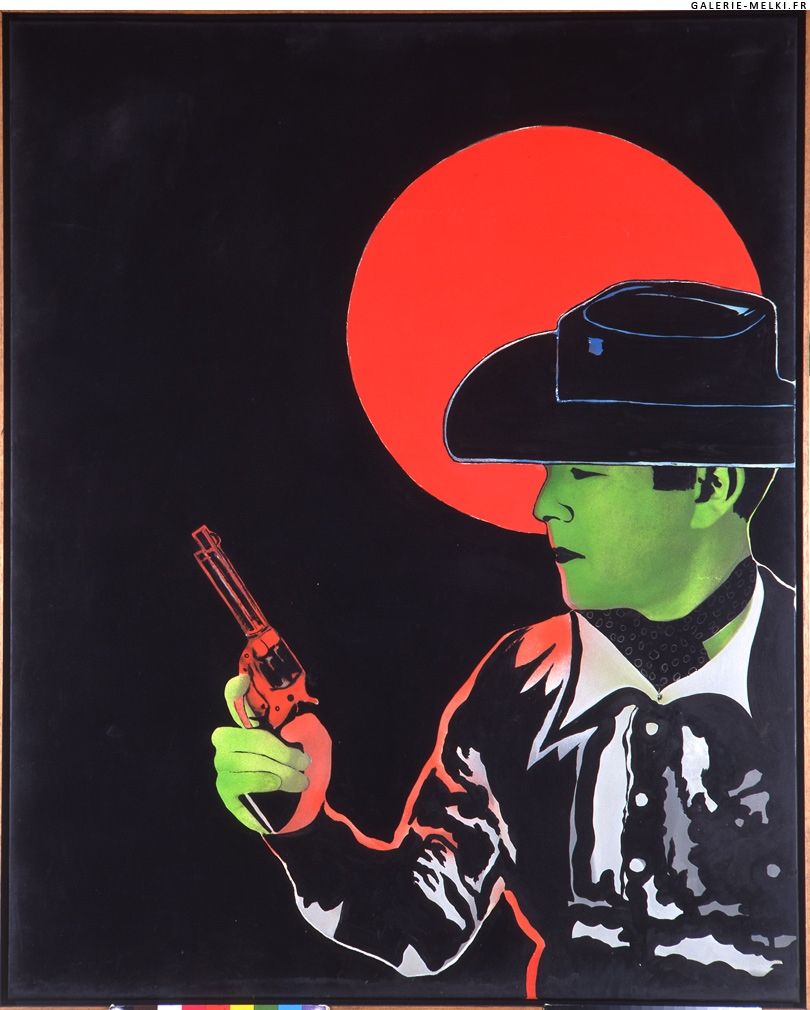The image depicts an illustration of a man dressed as a Hollywood cowboy with green skin. He faces towards the left, holding a pistol that reflects red, his finger poised over the trigger guard, and other fingers gripping the holster behind the gun's handle. His thumb, notably red, wraps around the other side. The man is adorned in a black shirt with white accents around the collar and chest, paired with a black and white long-sleeved element. He also sports a black tie with polka dots or possibly a scarf around his neck, and completes his attire with a black cowboy hat trimmed in white. Behind him, a red sun is partially obscured by his hat, set against a stark, completely black background. In the top right corner of the image, the text "galerie-melki.fr" can be seen.